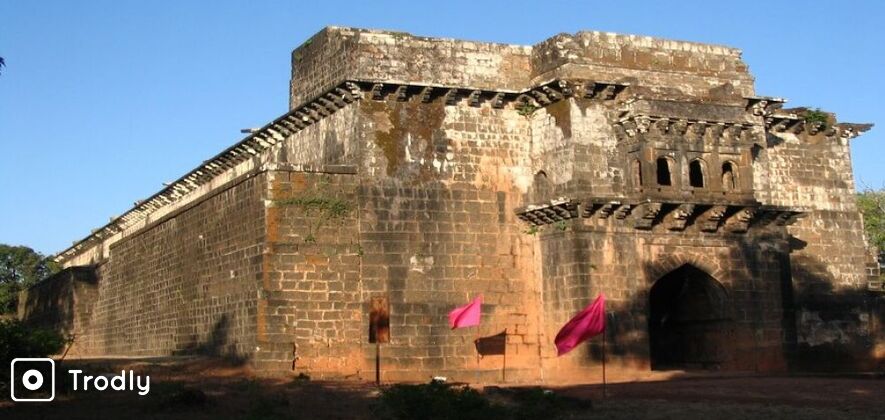This image depicts a weathered, ancient structure resembling a castle or temple with a distinctly broad, horizontal and rectangular shape. The building, primarily made of brick or concrete blocks, exudes an air of historical grandeur and antiquity, evident through its multiple shades of dark tan at the bottom, transitioning to white at the top, with distinct stripes of dark tan interspersed throughout. The very center boasts an arched doorway, accentuated by an additional rectangular structure that extends upwards from the top center of the building.

Outdoor elements emphasize the building’s serene environment, including a clear, blue sky and a backdrop featuring trees, suggesting it is situated amidst or adjacent to nature. The ground appears sandy, contributing to the South American castle-like vibe.

Foreground details include artistic features such as four flags fluttering near the structure. These flags are of varying colors: magenta, a dark indiscernible hue, pink and magenta, and a vibrant mix of orange, black, and yellow. Text on the left-hand side of the image spells out "TRODLY," accompanied by a small camera frame icon. Additionally, plant growth over parts of the building adds to its aged and rustic charm, blending the ancient man-made edifice with the surrounding natural elements.